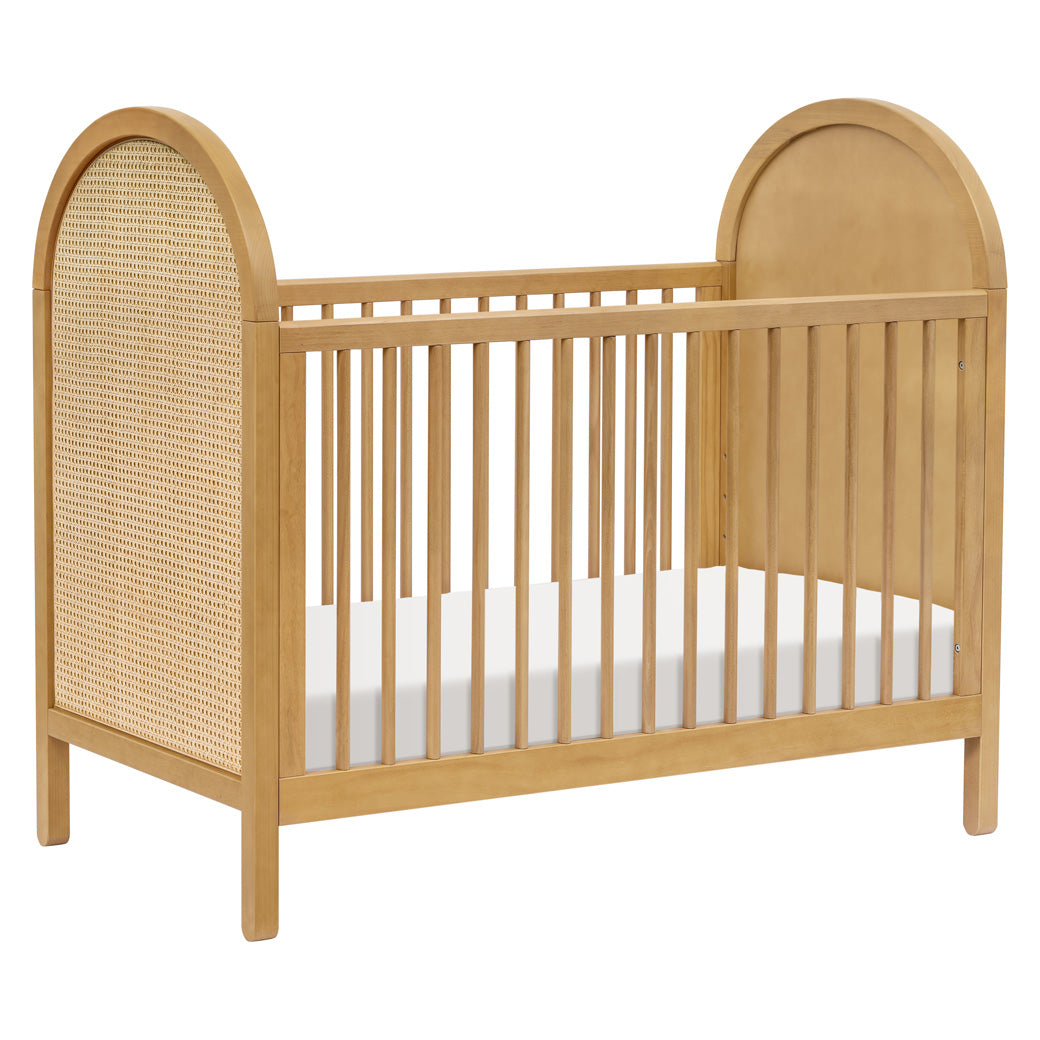This is a detailed product image of a baby's wooden crib, designed with safety and simplicity in mind. The crib features a light-colored beige wood finish with each end arching gracefully at the top, reminiscent of a classic design. One end is adorned with a rattan or wicker inlay that adds a touch of texture and elegance. The sides of the crib are constructed with sturdy wooden slats arranged vertically, ensuring the baby stays securely inside. Unlike many cribs, these sides do not appear to be adjustable. The crib stands on square legs, which, being fairly low to the ground, might require you to stoop to place or retrieve the baby. Inside, there's a pristine white mattress that fits snugly within the frame. The overall design suggests it could be an affordable, yet stylish and functional choice for budget-conscious parents. The photo focuses solely on the crib against a plain background, highlighting its features without any distractions.